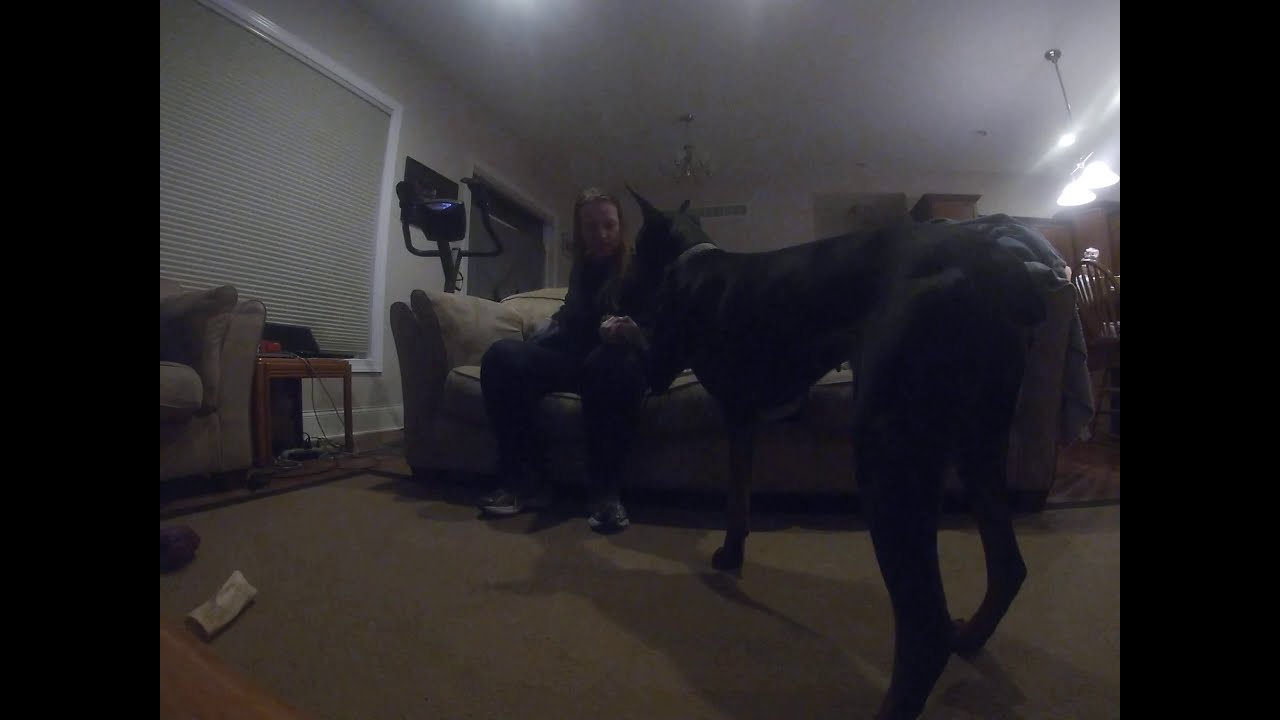In this detailed living room scene, a man with shoulder-length hair is seated on a beige couch, dressed in black pants, a black shirt, and sneakers. A large black dog with pointy ears is standing attentively in the center of the room, with one paw gently resting on the man's knee, exuding a calm demeanor. The room features brown carpet and another beige couch peeking in from the left side of the image. A large window with white borders and closed blinds is also on the left, suggesting it might be nighttime. Additionally, an exercise bike is visible behind the man. To the right, there is an adjoining area that appears to be a kitchenette or dining room, showcasing brown dining chairs, cabinets, and various lighting fixtures. Several lamps on the right cast shadows and reflections across the scene, adding to the cozy ambiance.